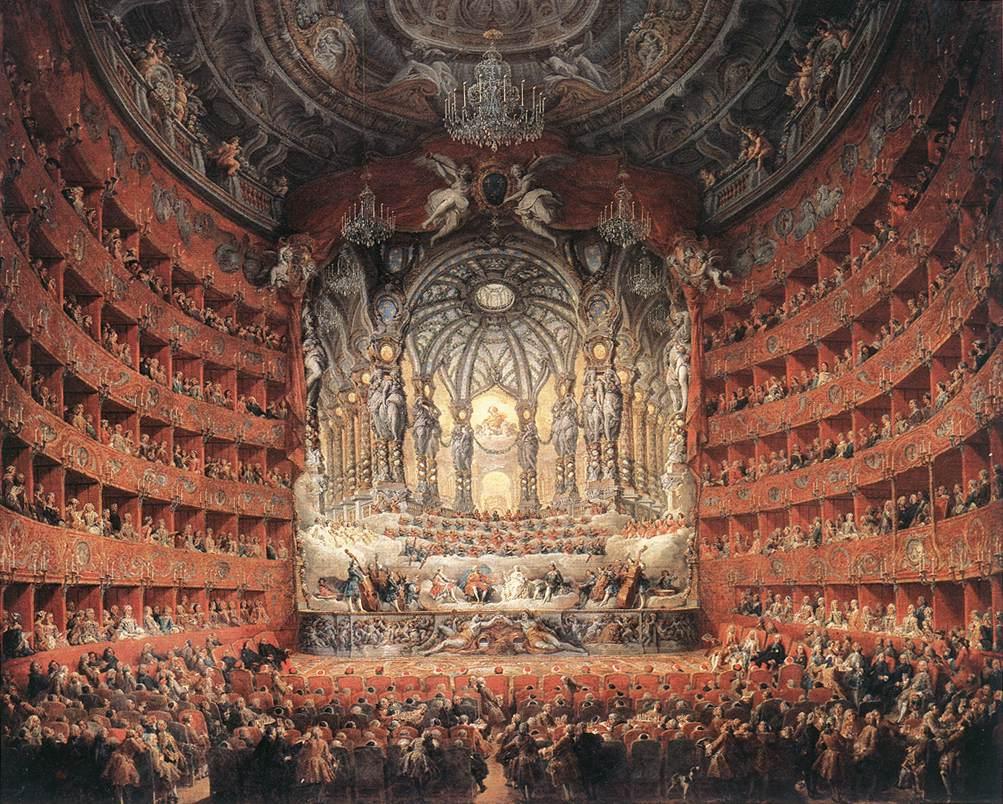The image is a highly detailed painting depicting the interior of a grand Baroque-style opera house. The setting is extraordinarily elaborate, with an overwhelming sense of ornate architecture and rich gold, red, and warm hues dominating the scene. In the center of the image is a stage, which is itself an intricate focal point, adorned with mythological figures and set against a backdrop featuring columns, clouds, and a cupola suggesting a heavenly tableau. The stage is flanked by numerous balconies—five levels on either side—each crowded with spectators in red box seats. The floor area is also packed with rows of chairs filled with audience members. The ceiling is adorned with chandeliers and ornate painted designs, adding to the luxurious ambiance. This opulent depiction is committed to capturing the lively atmosphere of a concert or opera performance, with every seat occupied and every corner filled with elaborate decoration, conveying the grandiosity of the event.